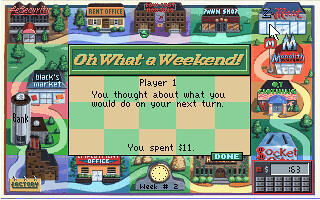A small rectangular video game screenshot is depicted, bordered completely by various buildings representing different establishments. The top, bottom, left, and right sides of the image showcase a diverse array of structures including a rent office, pawn shop, convenience store, fast food restaurant, bank, post office, market, and factory. In the bottom right corner, there is an icon of a calculator, while the bottom center contains an icon of a clock. Centrally located within the screenshot, a small square with a green border at the top displays the text "Oh, what a weekend" in yellow. Beneath this, a yellow and green checkerboard pattern fills the background, with black typeface reading: "Player One, you thought about what you would do your next turn, you spent $11."